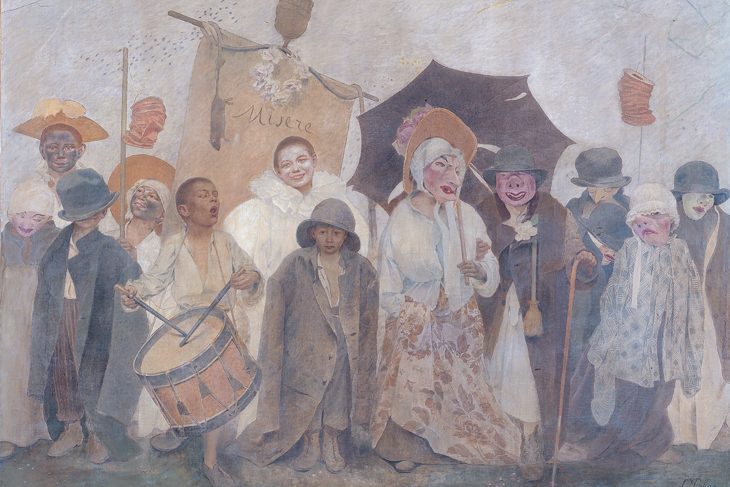This image is an intriguing, hand-painted illustration characterized by its muted, almost gray-washed colors. It depicts a diverse group of figures, including children and grotesque, monster-like characters, suggesting a possible Halloween or masquerade theme. At the center, a boy energetically beats a drum. Surrounding him are various children dressed in oversized, adult clothing: one boy wears a long coat and sun hat with his face obscured by blue ink, another dons a top hat and a too-large jacket, while a third has black marks all over his face. There is also a child with an angelic appearance in a fluffy white outfit reminiscent of a clown's ruffled collar. Offset to the side are more disturbing figures: one person has a pig's face, another a wildly distorted visage, and two others in the background wear elaborate hats, their faces also heavily disfigured. An ominous character with an intriguing face dons a dress and sun hat, standing slightly apart. Additionally, the scene includes peculiar details like a brown umbrella and a piece of parchment paper with a rat hanging by its tail, enhancing the unsettling atmosphere of the image.